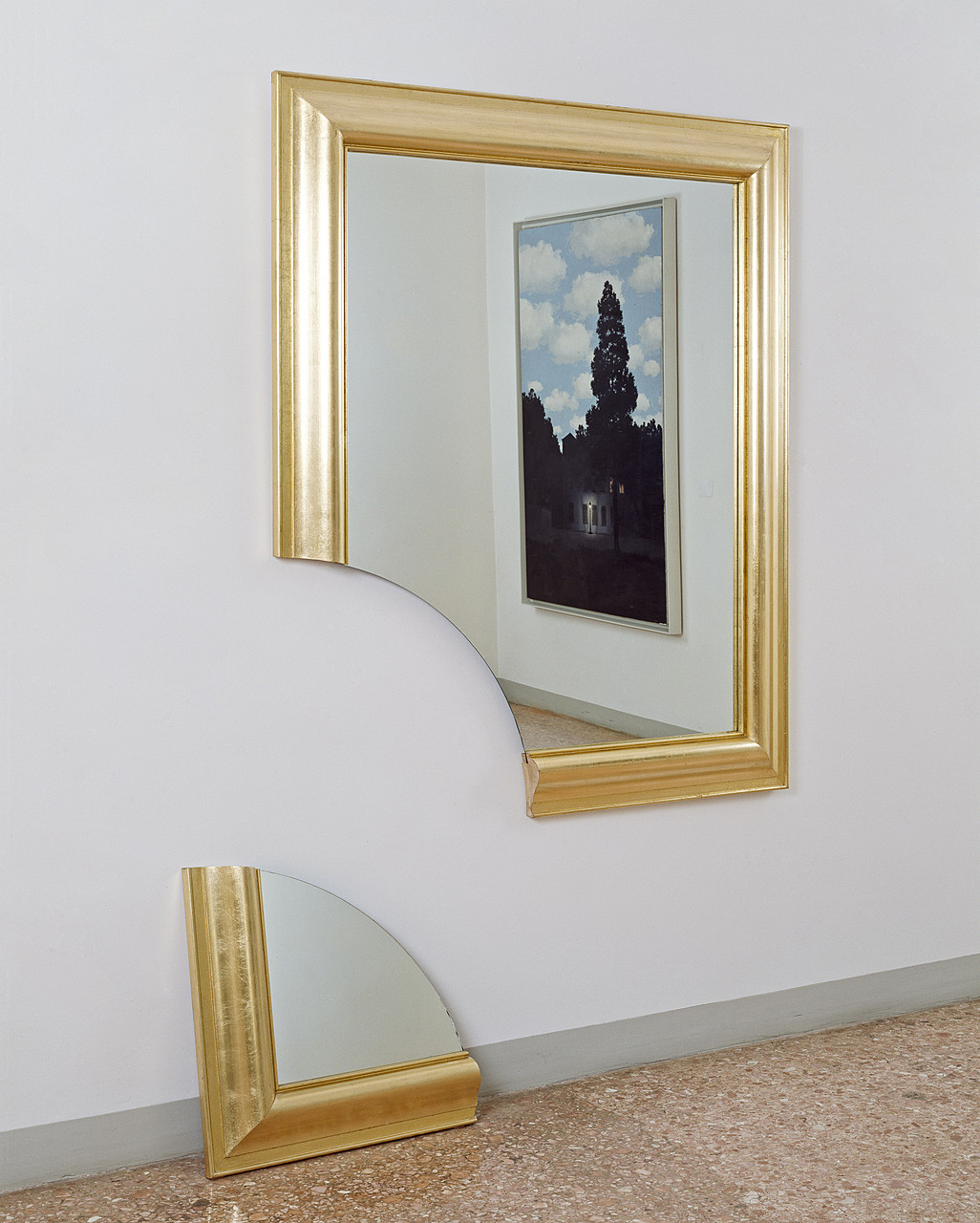The image depicts an intricate scene with a primary focus on a golden-framed painting or mirror mounted on a gray wall. The frame, painted in a rich gold hue, encloses the artwork in a perfect square shape. However, there's a distinct detail: the bottom left corner of the frame has a smooth, circular cut, resulting in that piece lying on the light-brown, stone-speckled linoleum floor beneath it. The cut-out segment is placed against the gray wall, which fades into a darker gray trim at the bottom. The content of the artwork inside the frame presents an outdoor scene, featuring a house, a large tree, and a sky dotted with clouds. The overall setup suggests a curious contrast between the intact and fragmented, drawing attention to the unusual circular separation at the bottom left of the gold-framed artwork.